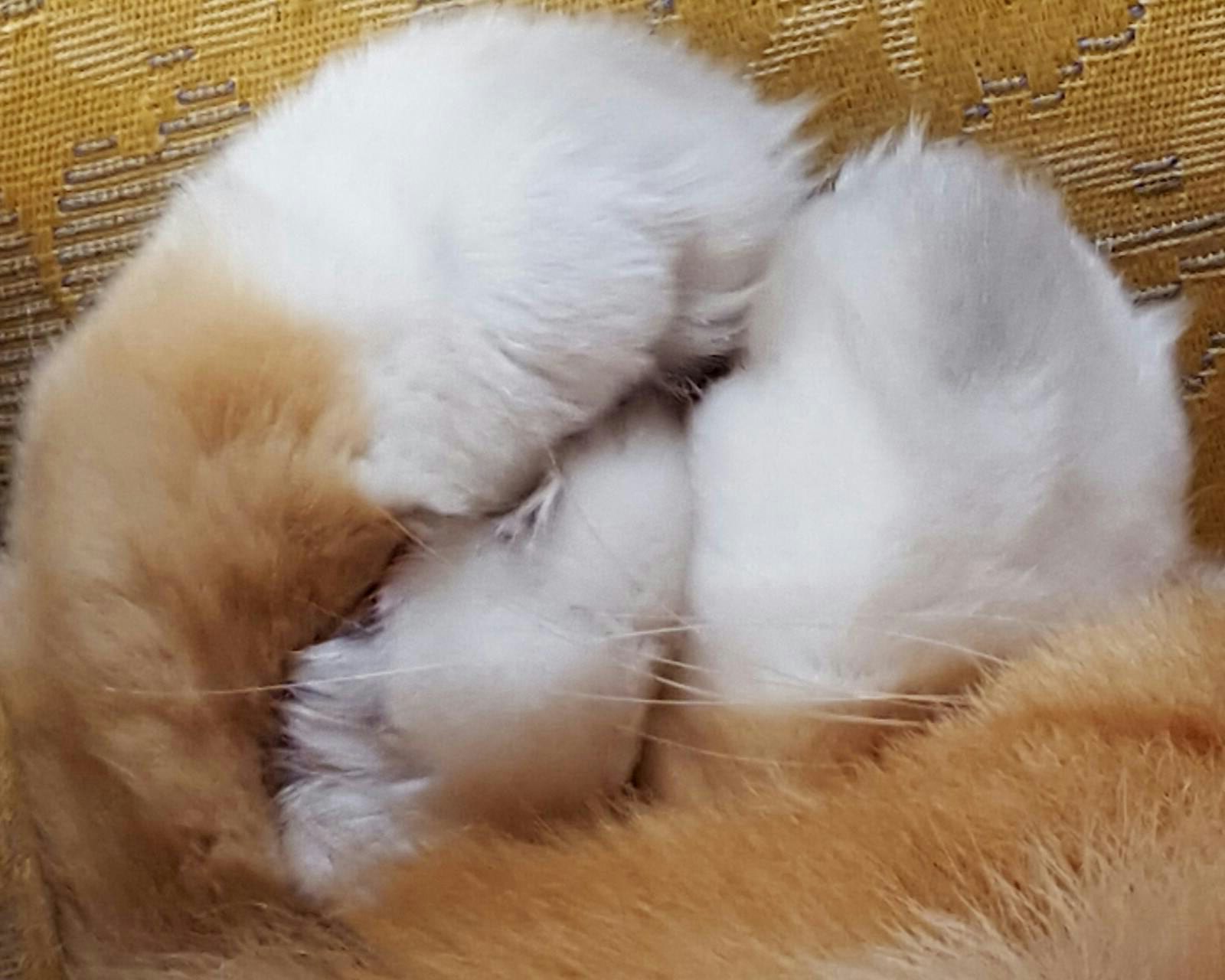The detailed close-up photograph captures an adorable orange and white cat, whose fluffy white paws and tail are prominently featured. The paws are curved and snug against each other, with subtle glimpses of the cat’s nose and white whiskers peeking through. The white fur on the paws and tail contrasts beautifully with the cat's light brown and orange fur, which has a sandy hue with faint lines. The background adds a soft, textured touch with its beige hue and subtle lines. Additionally, the cat is lying on a fabric with an orange and gold tapestry pattern, enhancing the cozy and warm ambiance of the scene.